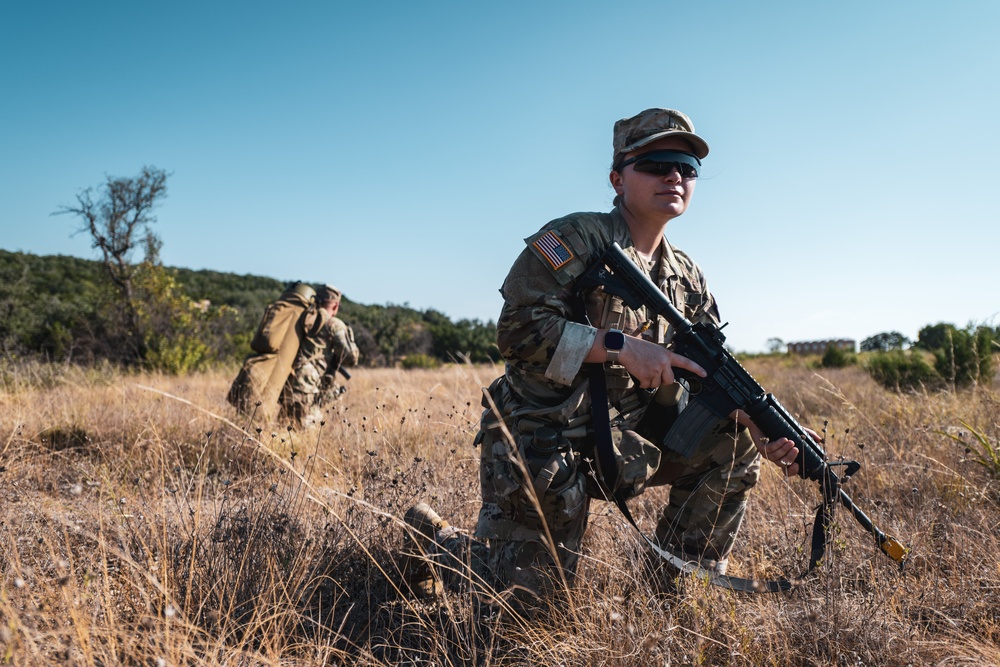In this detailed photograph taken on a sunny, cloudless day with a bright blue sky, we see a female soldier, likely a member of the army or National Guard, kneeling on one knee in a dry, brown grassy field. She is wearing a typical soft army hat with a brim, sunglasses, and a uniform adorned with an American flag patch on her right shoulder. She is equipped with a digital watch and holding an AR-15 with a sling. Behind her, another soldier can be seen carrying a large brown backpack, facing away from the camera towards the horizon. The background features a tree-lined hill with sparse shrubs and trees to the right, and a taller, leafless tree closer to the foreground. On the far horizon, a row of approximately ten portable toilets suggests that the area is a training ground for military drills or reconnaissance activities. The meticulous details and clear sky imply that this is an outdoor training exercise.